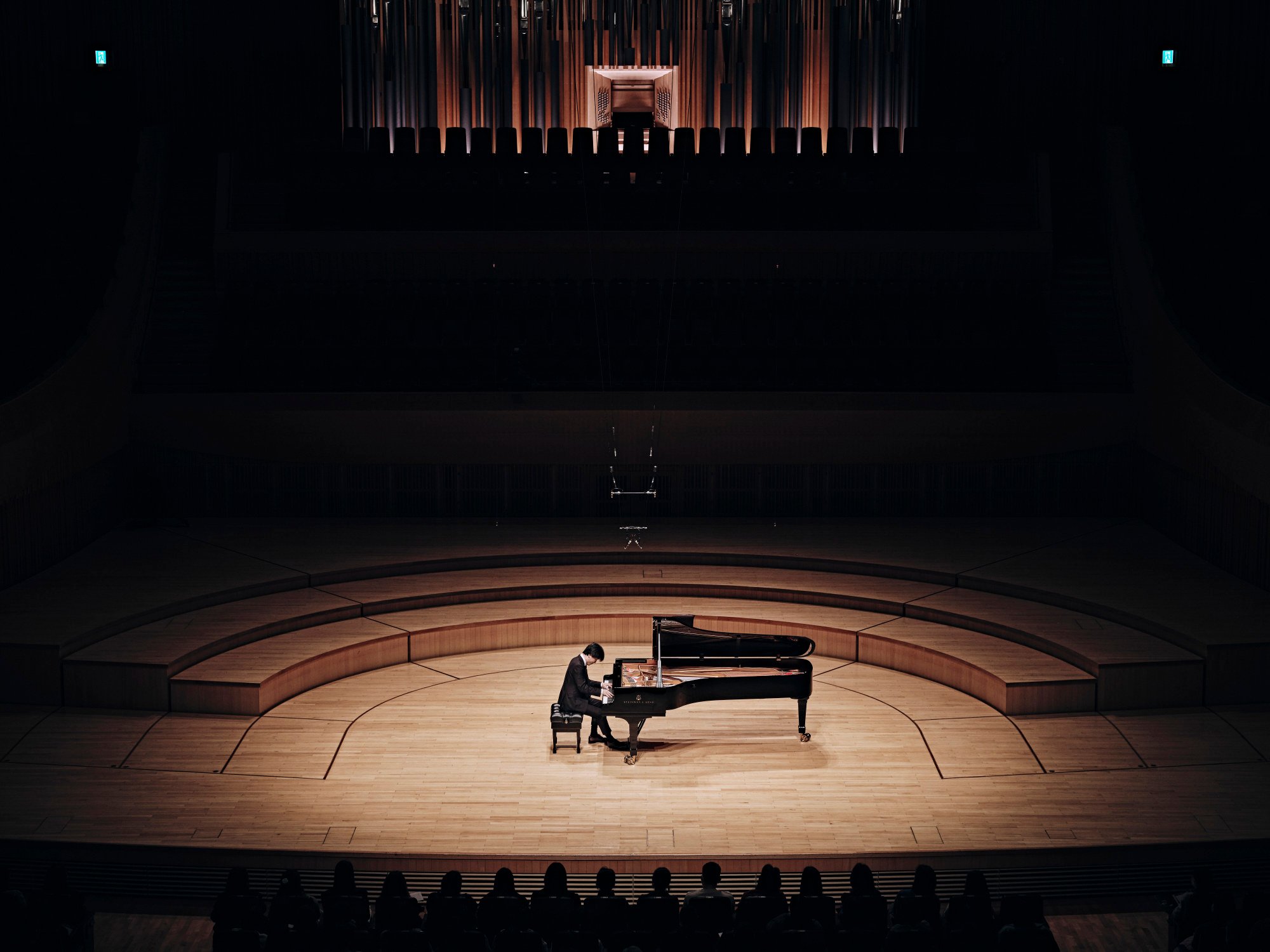The photograph captures a solitary pianist, a slim, middle-aged Caucasian man, elegantly dressed in black, seated on a black bench as he performs on a grand piano. The piano's lid is open, revealing its polished, impeccable craftsmanship. The stage is expansive, featuring U-shaped, brown-colored risers which encircle the performer, and wooden architectural elements that enhance the ambiance. A singular, intense spotlight illuminates the pianist and his instrument, creating a sharp contrast with the predominantly dark background of the auditorium. The setting appears to be an orchestra hall, with modern wooden fixtures and black curtains that hang high above. Though the room is dimly lit, the first and possibly the second row of the audience is faintly visible, seated in shadows, intently observing the performance. Scattered small lights, possibly exit signs, make subtle appearances in the otherwise darkened hall, contributing to the overall somber and focused atmosphere of the concert.